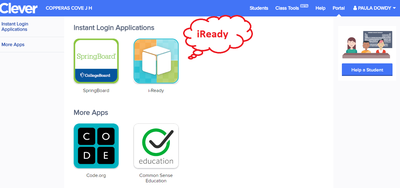This is a detailed screenshot of the Clever website interface, prominently featuring the Clever logo in the top left corner. Below the logo, the page is titled "Compass, Cobb J.H." The navigation bar contains buttons labeled "Students," "Class Tools," "Help," and "Portal." On the top far-right, the user's profile with their name is displayed. On the left-hand side of the screen, there are two main sections labeled "Important Login Applications" and "More Apps."

Under the "Important Login Applications" section, two instant login applications are listed: "Springboard" and "iReady." The "iReady" icon is marked with a red speech bubble containing the text "iReady." The "More Apps" section showcases two additional applications: "Code.org," represented by four black squares each containing a letter forming the word "CODE," and "Common Sense Education," which is depicted by a green circle with a black checkmark on a white background. The overall page has a simple white background, complementing its clean layout.

On the right side of the screen, there is a section labeled "Help a Student," featuring a blue button with the text "Help Student." Beyond this, the page is primarily white, maintaining a straightforward and user-friendly interface.